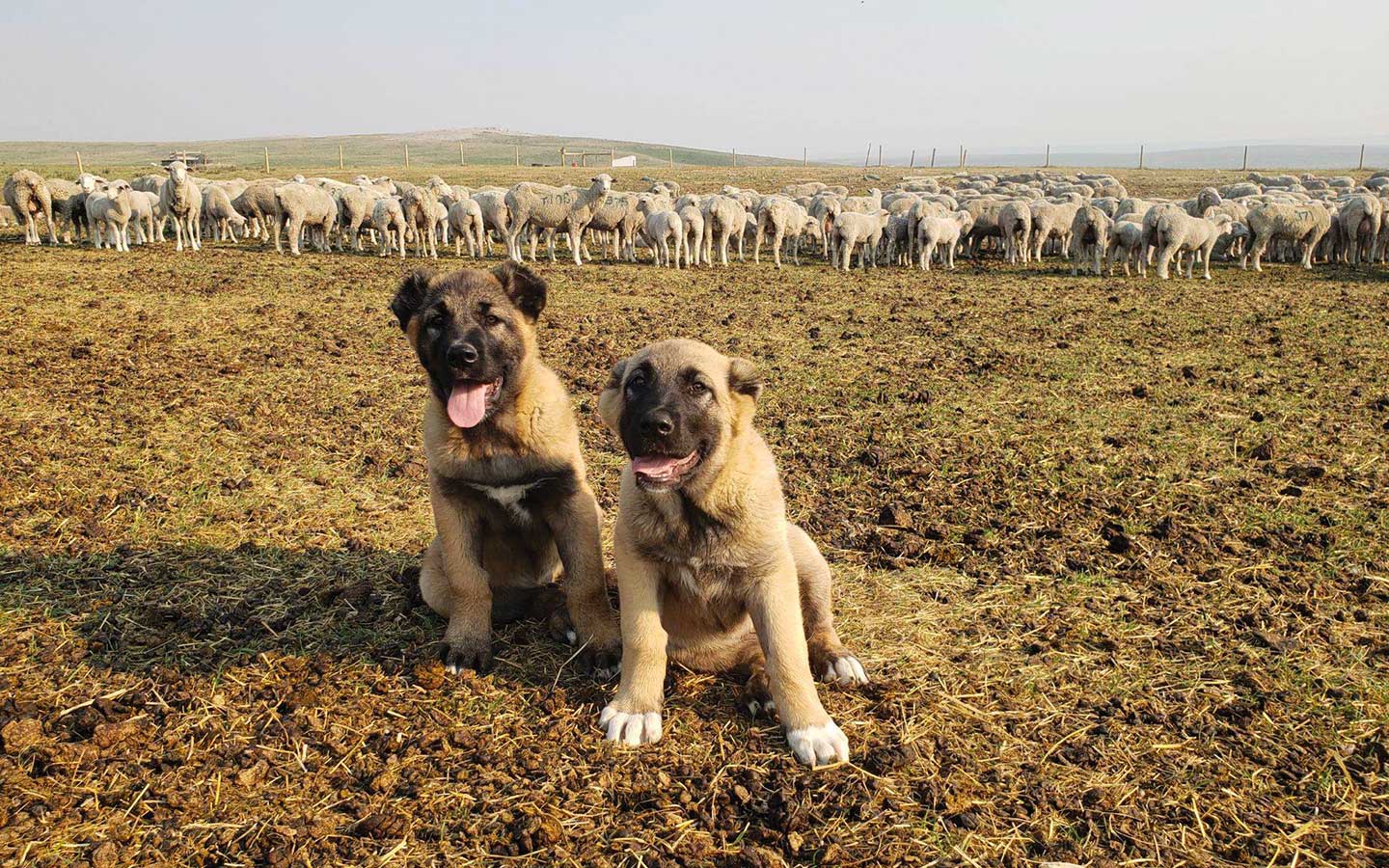In the outdoor photograph, a large grazing plot extends across the landscape, showcasing heavily grazed grass underfoot. At the forefront and center of the image, two small puppies, likely herding dogs, pose adorably for the camera. Both have tan fur with distinctive dark facial features and their mouths are open, tongues lolling out. The puppy on the left has dark markings along the edges of its paws, ears, and chest accompanied by a small white V of fur. The puppy on the right is quite similar but has white markings at the tips of its paws. 

Directly behind the puppies, a herd of sheep is visible, grazing peacefully. The open plain continues into the distance, where a fence marks the boundaries of the grazing area. Beyond the fence, another hill rises, adding depth to the scene. The sky above is light and overcast, perhaps shrouded in fog or smog, lending a muted tone to the landscape. In the far distance, another low, darker colored rolling hill contrasts with the otherwise pale sky, completing the tranquil rural setting.